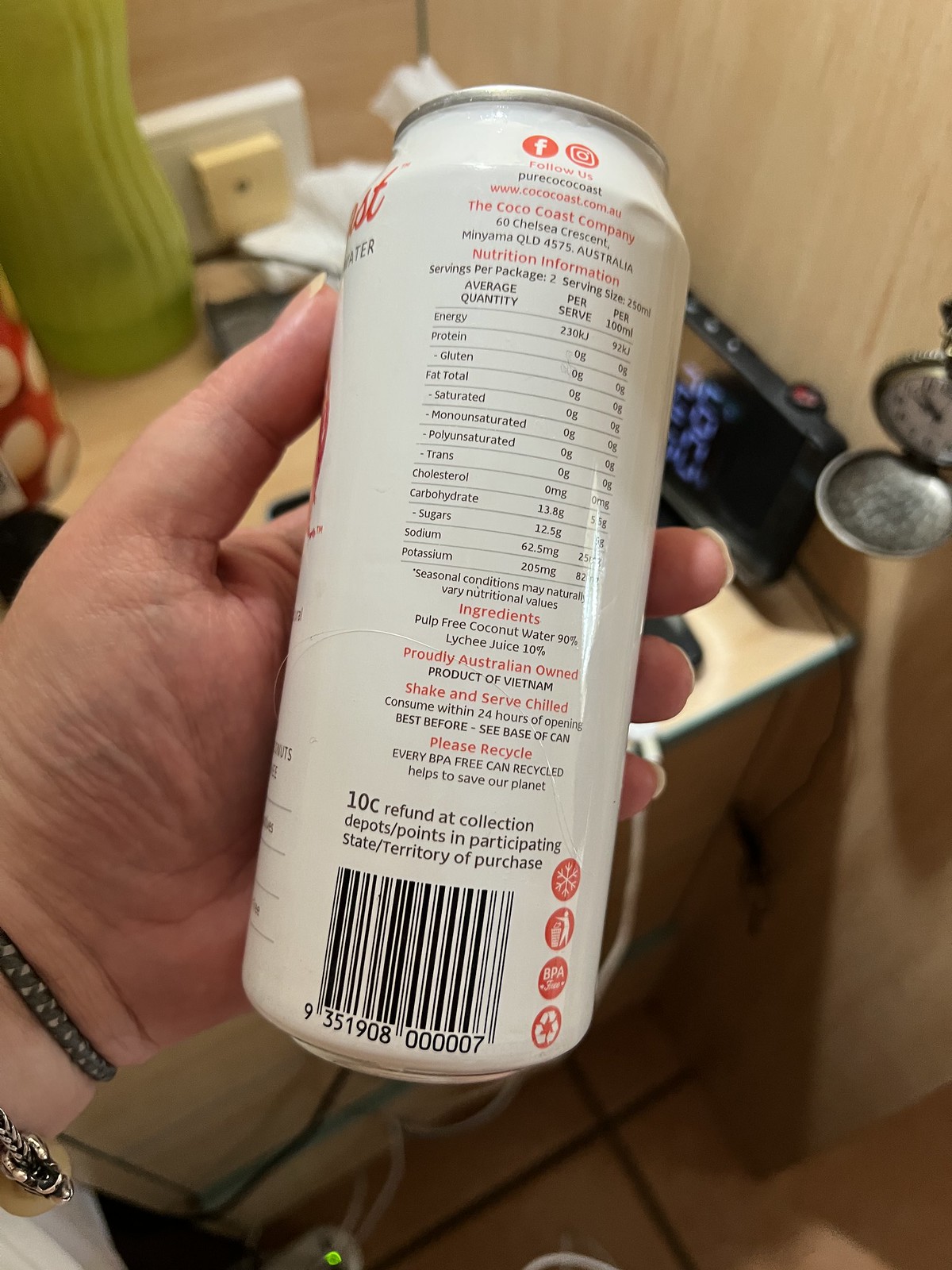A person stands in a room holding a white can with an intricate design featuring various symbols and information on its label. The label’s top section showcases social media icons for Facebook and Instagram with the prompt "Follow us," followed by the brand name "Pure Cocoa Coast" and the website "www.cocoacoast.com.au". The address "60 Chelsea Crescent, Minyama, QLD 4575, Australia" is also listed, identifying the company's location.

Moving down, the label displays comprehensive nutritional information, indicating the can contains two servings, followed by a detailed breakdown of nutritional content—energy, protein, gluten amount, and total fat, which is further divided into saturated, monosaturated, polyunsaturated, and trans fat. Additional nutritional data includes cholesterol, carbohydrates (broken down into sugars), sodium, and potassium.

Below this nutritional data, the ingredients are listed as 90% pulp-free coconut water and 10% lychee juice. The label notes the product is probably Australian-owned but manufactured in Vietnam. Directions advise consumers to "Shake and serve chilled," and to "Consume within 24 hours of opening." It also notes to "See the base of the can for the best before date" and encourages recycling with the message, “Please recycle. FEPPA free can, recycle helps to save our planet.”

Further down, a recycling refund notice states a 10-cent refund is available at collection depots in participating states or territories. A barcode is positioned towards the bottom, marked with the number 935190800007, flanked by four symbols: a snowflake on a red background, a man near a trash can, a label indicating "BPA free," and a recycling symbol. This detailed representation encapsulates the product's branding, nutritional facts, origin, and environmental considerations.